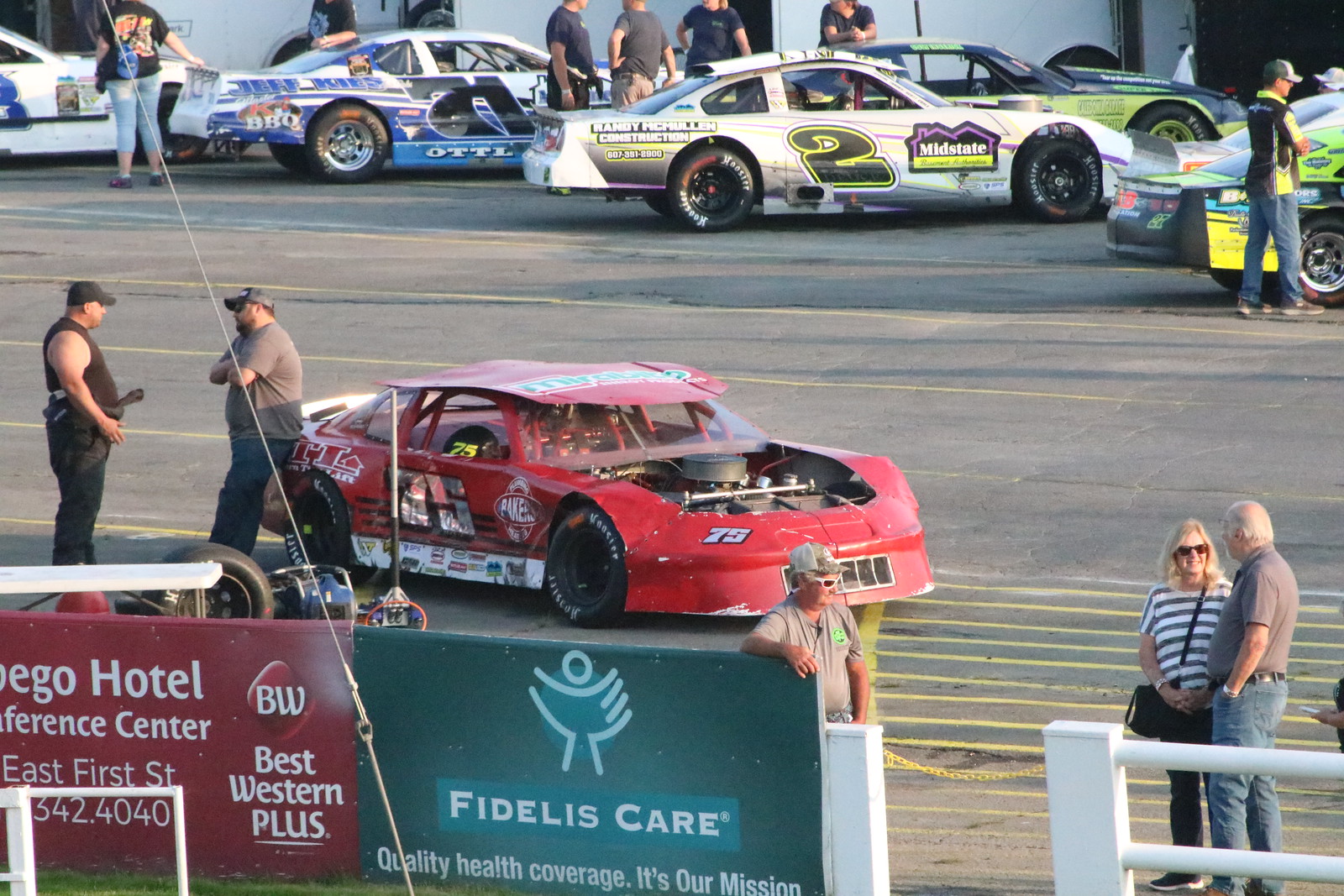The image depicts a bustling pit area at an outdoor racetrack with at least six brightly colored race cars, all showcasing various sponsorships. Dominating the foreground is a red race car, marked with the number 75, with its hood removed and temporarily placed on the roof, revealing a red roll cage inside. The car lacks a driver, and a heavyset man leans against its rear quarter panel, engaged in conversation with another heavyset man in a black tank top and hat. Around them, pit crew members, racers, and staff tend to the other cars, some of which display numbers like 2, 71, and 78, with one car featuring the word "Mid-State." Visible in the background, behind a white fence, are sponsorship banners, including a prominent Fidelis Care sign promoting quality health coverage and a maroon Best Western Plus Conference Center sign. The activity and interaction among the people and the detailed sponsorships create an energetic atmosphere typical of a racetrack pit area.